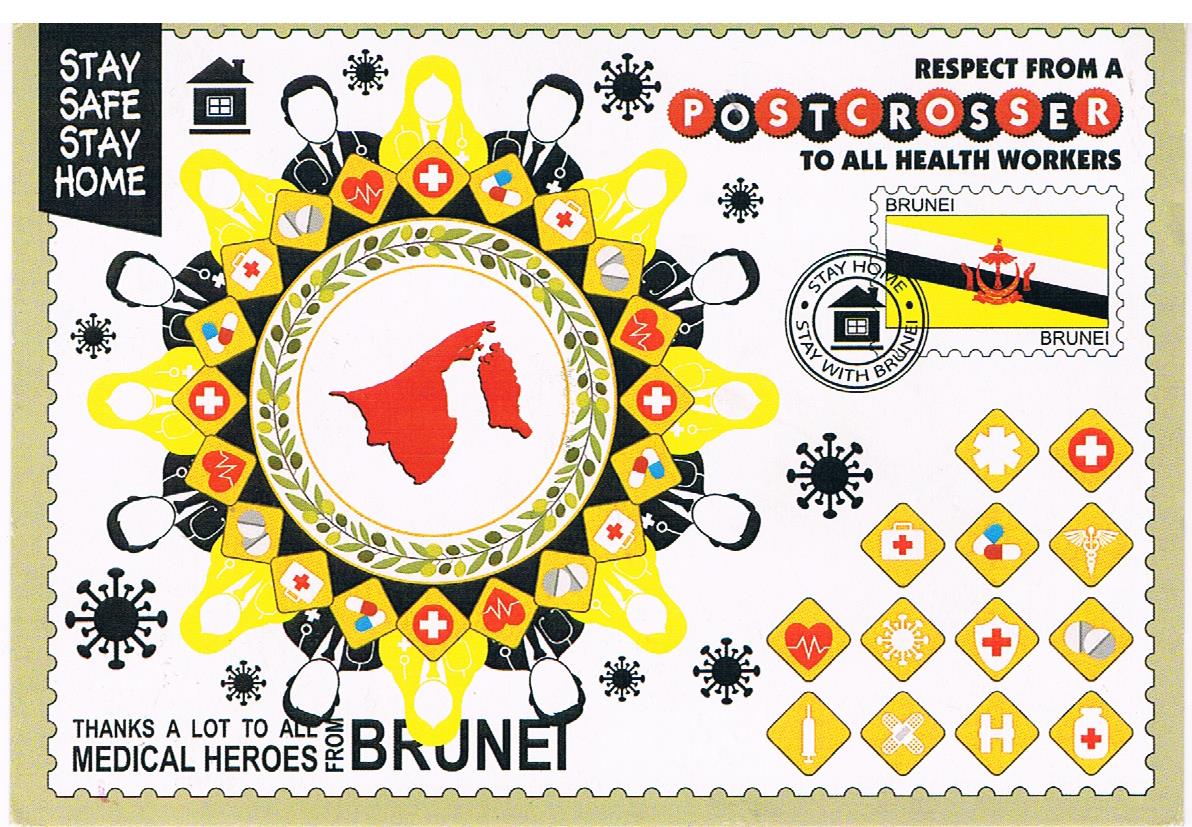This image resembles a postcard or an elaborate thank-you card dedicated to medical professionals. The central feature is a large, circular illustration with a red outline of Brunei at its center, surrounded by a decorative vine pattern. Around the circle are drawings of medical professionals—doctors and nurses—depicted in blue, with blank faces and detailed hairstyles, seated around what appears to be a circular table covered with various medical items illustrated on yellow squares. These items include pills, medical charts, and Red Cross symbols.

Positioned in the upper right corner, blue text on a white background reads, "Respect from a postcrosser to all healthcare workers," with alternating red and blue text circles below saying "postcrosser." Below this, another message in blue letters states, "to all our health workers," next to what appears to be a postage stamp from Brunei, incorporating a yellow hue with a white and blue vertical banner bearing a symbol of Brunei.

The top-left corner of the image features a white label on a blue background that reads, "Stay safe, stay home," accompanied by a drawing of a house. Additional images of germs and medical gear dot the background. The bordered edges of the picture are light brown with a ruffled white overlay, contributing to the decorative aspect of the card. Conclusively, the bottom of the image displays a heartfelt message in blue text that reads, "Thanks a lot to all medical heroes from Brunei," emphasizing the origin and the card's theme of gratitude and support during challenging times.